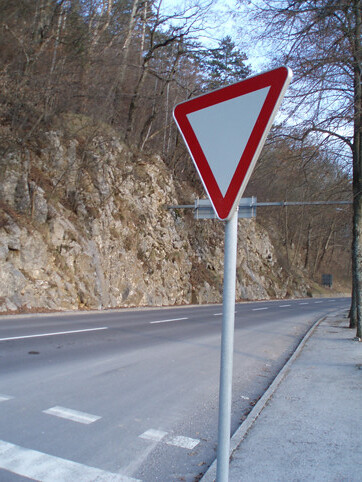In this image, there is a prominently displayed triangular traffic sign mounted to the right of the roadway. The sign has a white center with a red border and is affixed to a silver pole. It is situated near a sidewalk, adjacent to a two-lane road marked with white striping. On the far left side of the image, there is a landscape of high hills featuring a mix of brown rock and tall trees, some of which appear to be dead or dying. The setting suggests a mountainous or hilly area, indicating that the roadway is likely situated near a mountainous region. The triangular sign is the focal point of the image, emphasizing its importance in this scenic yet rugged environment.